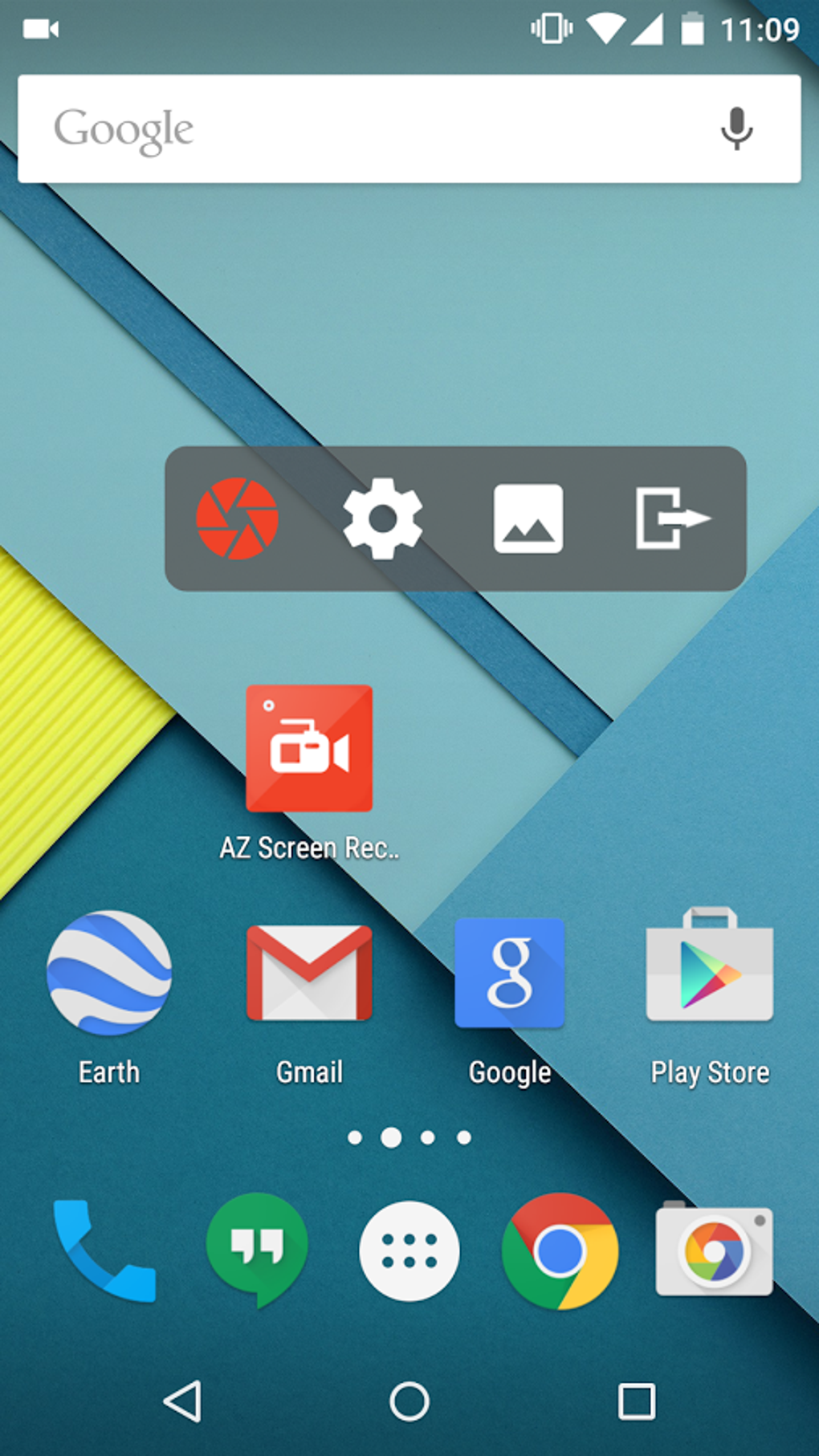This image is a screenshot of a smartphone's home screen featuring a blue-toned background transitioning from sky blue at the top to an aquamarine hue towards the bottom. Prominently displayed in the center-left is a small yellow triangle that resembles a piece of lined writing paper or a legal pad. At the very top of the screen, the status bar displays the time as 11:09, along with various notification icons.

Below the status bar, there is a Google search box, presented as a large, horizontally-aligned white rectangle. About halfway down the screen, there lies a light gray rectangle, which features several app icons. Among these icons are one red and three white symbols.

The bottom portion of the home screen houses two rows of familiar app icons. These include the blue phone icon, the Google Chrome browser icon, the Play Store icon, the Gmail app icon, and several others, providing quick access to frequently used applications.